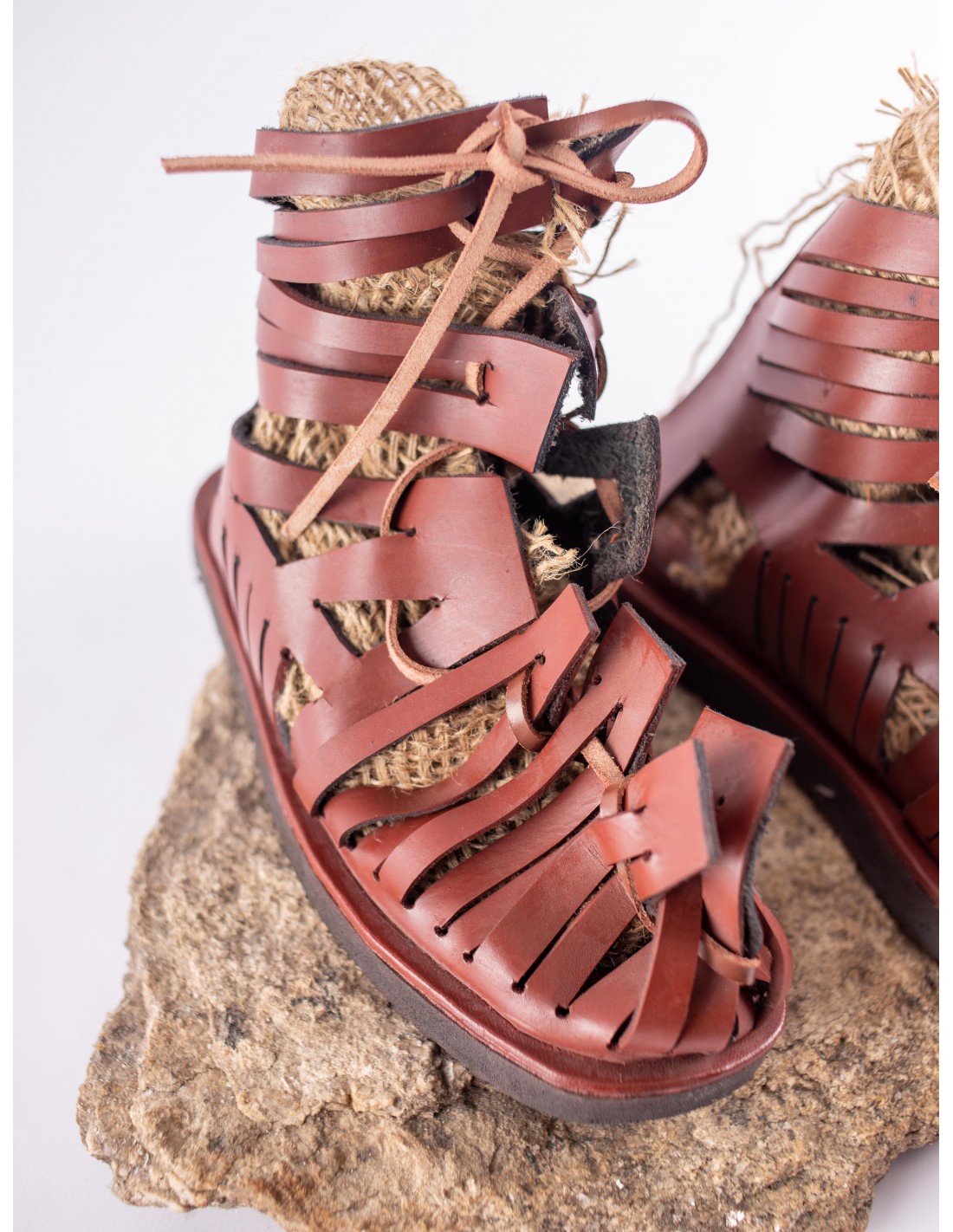The photograph showcases a pair of Roman-style sandals prominently displayed on a natural-looking brown rock. The focal sandal, placed slightly off-center to the left, is intricately designed with reddish-brown leather straps that extend up to the ankle, fastened by thin leather laces. The sandal features a woven, foot-shaped insert inside, demonstrating a fitted appearance. The interior of the sandal is black, contrasting with its red exterior. To the right, partially visible, is its matching pair. The overall setting is against a grayish backdrop, emphasizing the sandals and the rock they rest upon.